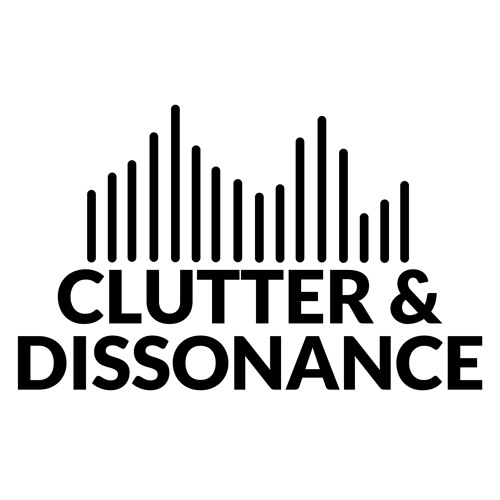The image features a minimalistic design dominated by a stark white background. Centered near the top is a black, wavy line resembling a graph or the bars of a signal strength indicator, with the pattern oscillating up and down in varying lengths. Below this graphic are two lines of bold, uppercase black text, reading "CLUTTER & DISSONANCE" in a clear, crisp font. The simplicity of the black and white color scheme, combined with the clean layout, suggests it could be a logo, possibly for a company or user creation, similar in style to a business brand like Cisco. The overall design exudes a sense of order amid chaos, hinting at themes of signal clarity and noise.